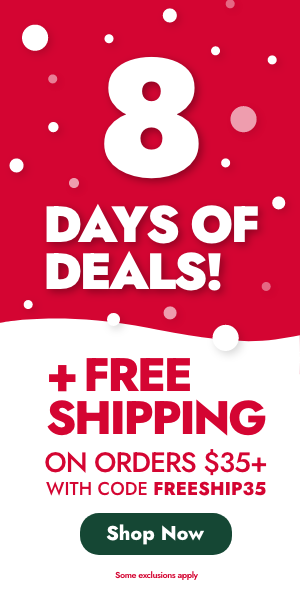A vibrant advertisement promoting a special sale event. The ad is rectangular and neatly divided into two distinct color sections. The upper half features a bold red background adorned with various sizes of white and pink dots, reminiscent of falling snowflakes. Dominating the center of this red backdrop is a large numeral "8" in white, indicating the "Eight Days of Deals" campaign. Below this, an eye-catching white text announces the promotion: "DAYS OF DEALS."

In the lower half of the ad, the background shifts to white, providing a sharp contrast for the red text that reads, "PLUS FREE SHIPPING." Further down, another line specifies: "On orders $35+ with code FREESHIP35." At the bottom center, a prominent horizontal black oval contains the call-to-action "Shop Now" in white letters, which are notably not capitalized. Beneath this button, fine red print informs viewers that "Some exclusions apply."

The harmonious blend of red and white hues, coupled with the use of festive dot patterns, suggests that this advertisement is geared towards the holiday shopping season, enticing customers with both significant deals and the added perk of free shipping.